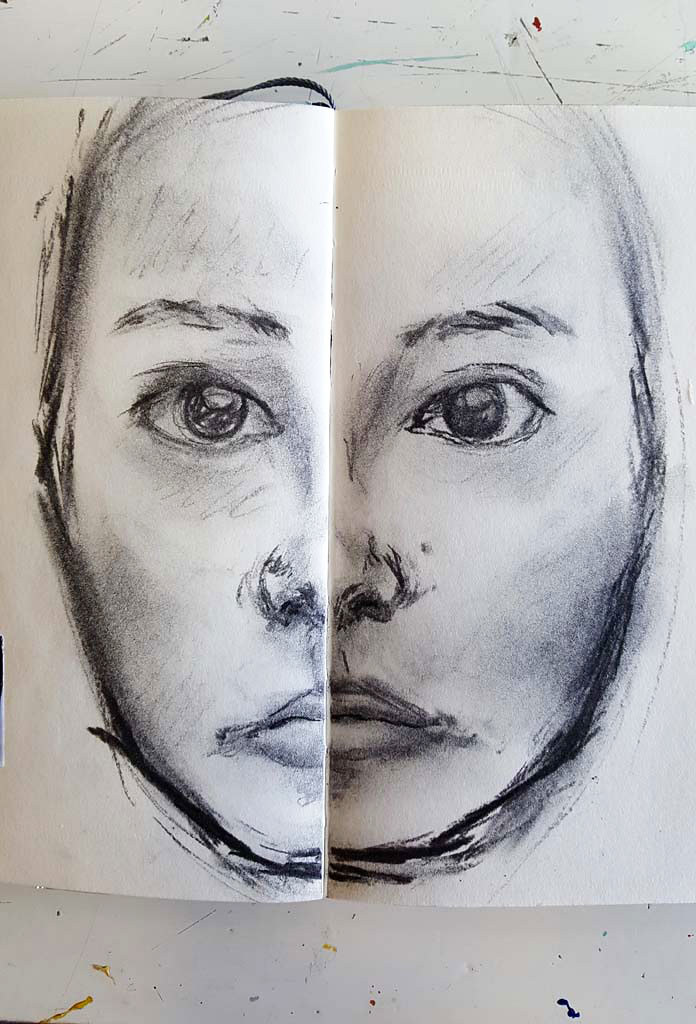The image features a detailed black and white sketch of a face drawn on a sheet of paper. The paper is oriented in landscape mode, almost squarely framed in the center of the image, with the upper and lower sections revealing a white background table marked with stray pen, pencil, or marker lines. There's a distinct vertical crease in the middle of the sheet, creating a slight upward bend resembling a small mountain shape.

The face in the sketch, devoid of any hair or neck, has an oval shape and is captured from just above the jawline to slightly below the top of the head. Thick lines, likely made with charcoal or a heavy pencil, outline the face. The eyes, large and staring directly at the viewer with pronounced irises, sit beneath well-defined eyebrows. Positioned centrally between the eyes is the nose, and below it, closed lips give the face a serious expression. The lips are noticeably fuller in the middle than at the edges, adding to the stern demeanor of the face, which appears to possibly depict that of a woman.